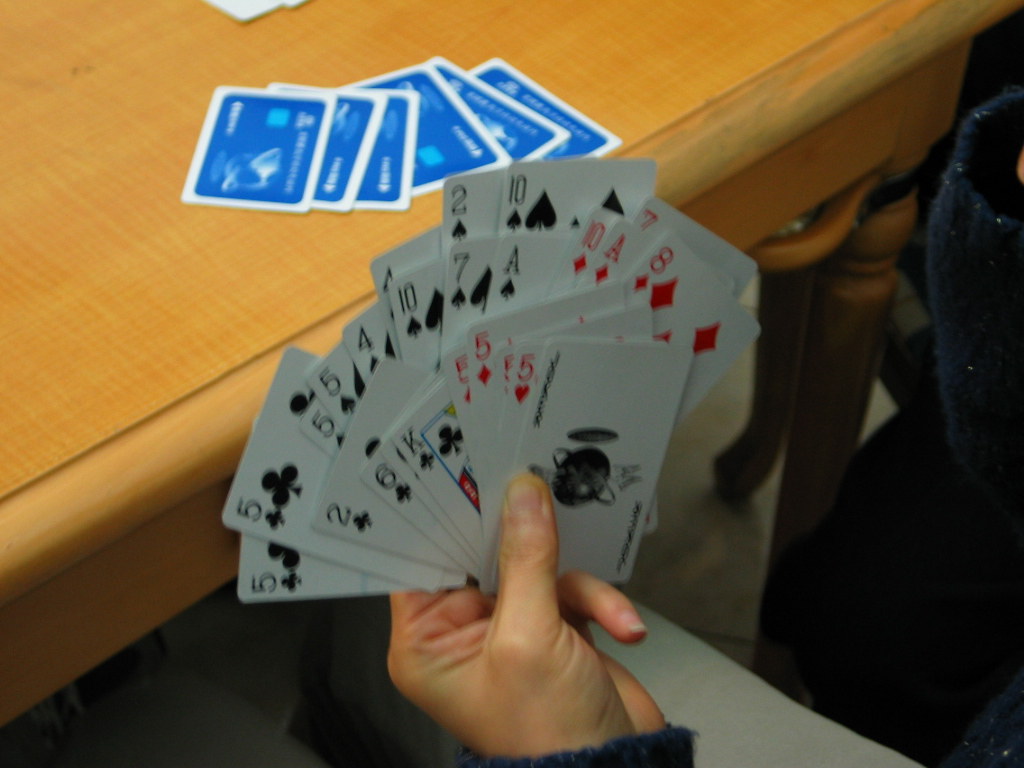The photograph captures a moment at a wooden table, which is an off light brown tan color, suggesting it is made of wood. In the upper left background, six playing cards are spread out face down on the table. The backs of the cards are royal blue and feature intricate designs.

In the bottom middle of the image, a person's left hand is holding a fanned-out deck of cards. The cards are partially visible, revealing a variety of denominations and suits: two 5 of clubs, a 5 of spades, a 4 of spades, another unidentified 4, two 10 of spades, a 2 of spades, a 7 of spades, an ace of spades, a 10 of hearts, an ace of hearts, an 8 of hearts, a 2 of clubs, a 6 of clubs, a king of clubs, a 5 of diamonds, a 5 of hearts, and a joker adorned with an image of a planet with a ring around it.

In the bottom right corner, the leg of the wooden table is visible, adding to the cozy, tactile feel of the scene.